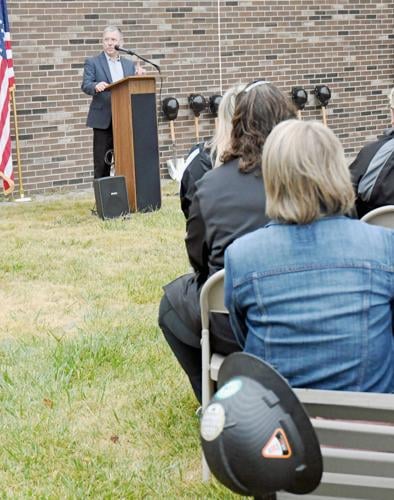The image depicts an outdoor ceremony set on a grassy area, featuring a man in a black suit, without a tie, speaking at a podium to an audience seated on metal folding chairs. The podium has a prominent microphone connected to a speaker to amplify his voice. He stands against a brown and black brick wall, with an American flag positioned to his right. Behind him, a row of shovels with black hard hats on top suggests a groundbreaking event, possibly a memorial service. The audience members, seen from the back, are listening attentively, with visible details including a jean jacket, a suit coat, and another black hard helmet hanging from a chair near the foreground. This scene evokes a formal and possibly commemorative occasion.